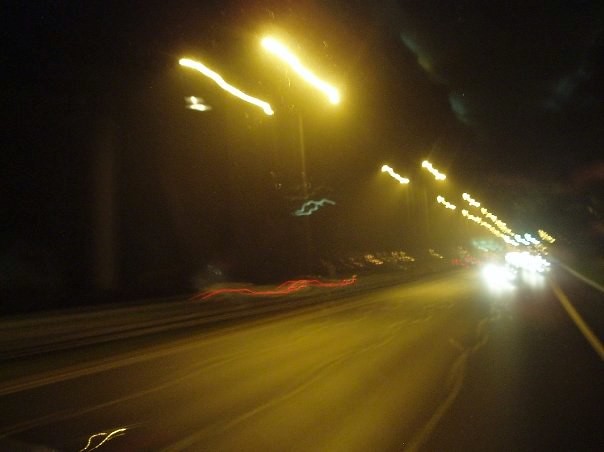The image captures a dynamic night-time driving scene, most likely photographed from a moving vehicle, possibly a dashcam or through a window. The photograph conveys a sense of motion with blurred, vibrant lights stretching across the frame. Red, yellow, and white streaks dominate, with the red lines suggesting taillights and the yellow and white lines appearing to stem from streetlights and possibly power lines above the roadway. There is a visible divider where the red squiggly lines converge, likely indicating vehicles moving in the opposite direction. The roadway itself is a large highway with multiple lanes; in some of these lanes, cars head towards the observer, their bright white headlights casting an intense glow into the distance. On the right side of the image, a painted white line hints at a small lane, perhaps for bicycles, while the left side features a hazy fence-like structure. Above, the long, thin streetlights extend far into the dark night sky, blending with the blurred lines below to create a surreal, frenetic urban landscape.